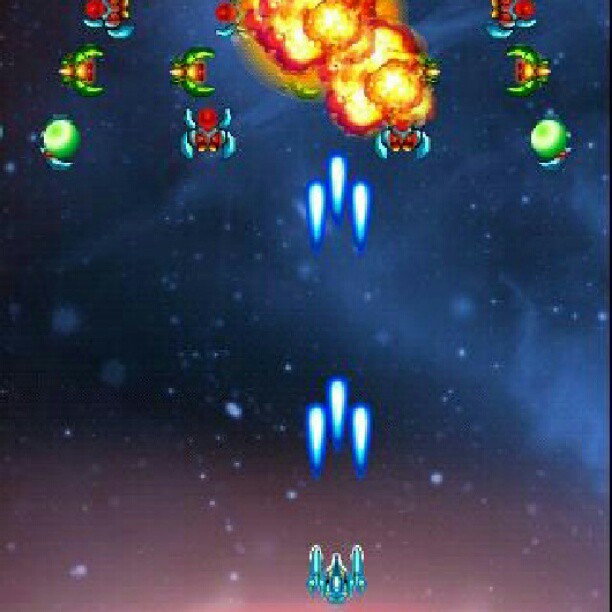The image resembles a vibrant and action-packed scene from a video game. The background gradates from navy blue at the top to light magenta at the bottom, creating a dynamic and colorful backdrop. Scattered across the entire image are small, blurry white dots, reminiscent of falling stars or space debris.

At the bottom of the image, a spaceship takes center stage, equipped with dual guns on each side and an additional one in the middle, launching three rays simultaneously. The scene vividly depicts two sets of these triple-shot rays piercing through the air.

Towards the top of the screen, several targets in various color combinations—green, green and red, and blue and red—are visible. One of these targets has been hit by the spaceship's rays, resulting in a spectacular explosion. Fiery bursts and flames erupt from the struck object, adding intensity and excitement to the scene. The detailed and vibrant artwork captures the essence of a thrilling intergalactic battle.